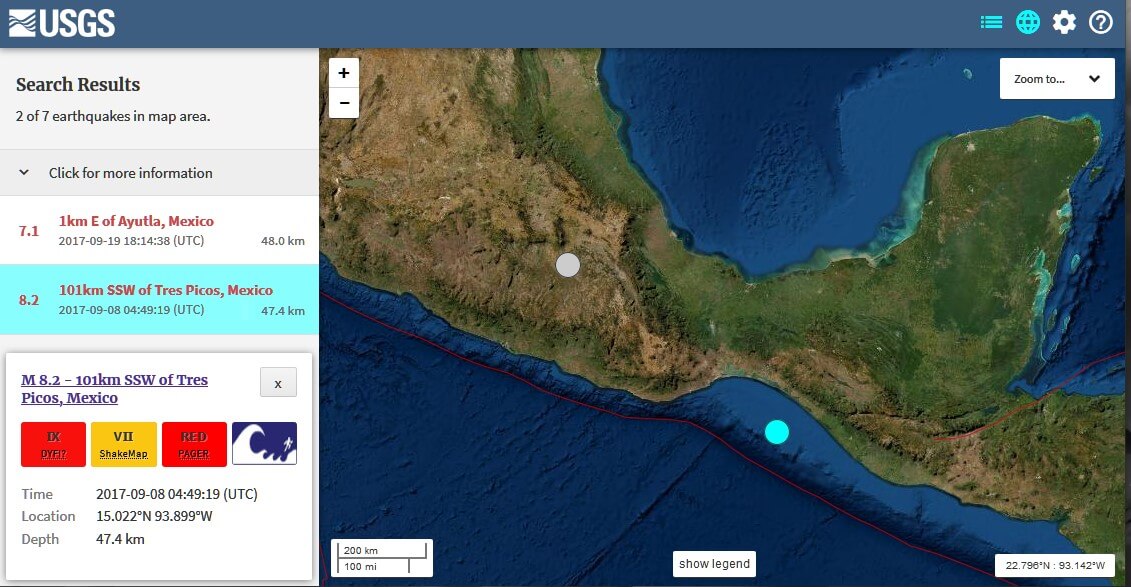This detailed map is sourced from the United States Geological Survey (USGS) website, displaying earthquake activity. Positioned on the right side of the webpage, the map highlights two significant earthquake events. One event is located approximately 1 kilometer east of Ayutthaya, Mexico, while the other is situated about 101 kilometers southwest of Tres Picos, Mexico. This visualization focuses on the lower part of North America, including the geographical regions of Mexico and potentially the southernmost part of California. The left panel of the webpage features search results, indicating that these two earthquakes are part of a larger data set consisting of seven total seismic occurrences in the area. The map provides a crucial tool for understanding and tracking seismic activity in this region.